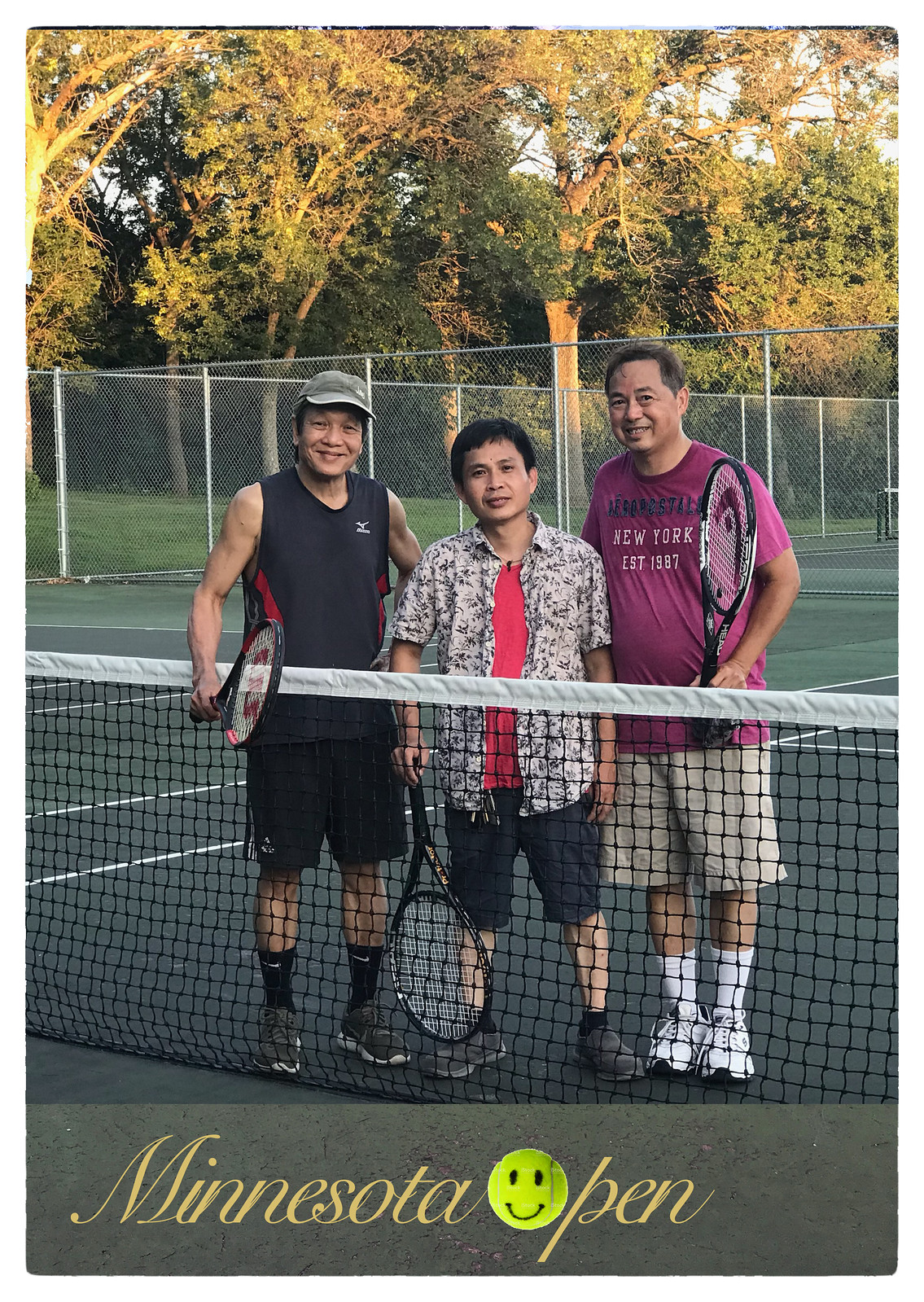The image depicts three men, presumably related, standing behind a tennis net on a green suburban court enclosed by high gray fencing. The background features trees with yellow leaves, hinting at an autumn setting. The man on the left, likely in his 40s, wears a black sleeveless shirt, black shorts, black Nike socks, gray shoes, and a ball cap. Holding a black-rimmed racket in his right hand, he stands next to a younger man in the middle, potentially the son. This younger man sports a white and black button-down shirt over a pink undershirt, black shorts, black socks, and black shoes, also holding a black-rimmed racket in his right hand. The man on the right, appearing to be the oldest and possibly in his 50s, is dressed in a maroon shirt with white text, beige shorts, white knee-high socks, and white tennis shoes, carrying a racket in his left hand. Beneath the image, a gray bar contains a caption reading "Minnesota Open" in yellow cursive font, with a tennis ball representing the "O". This humorous element underscores that they are amateur players.